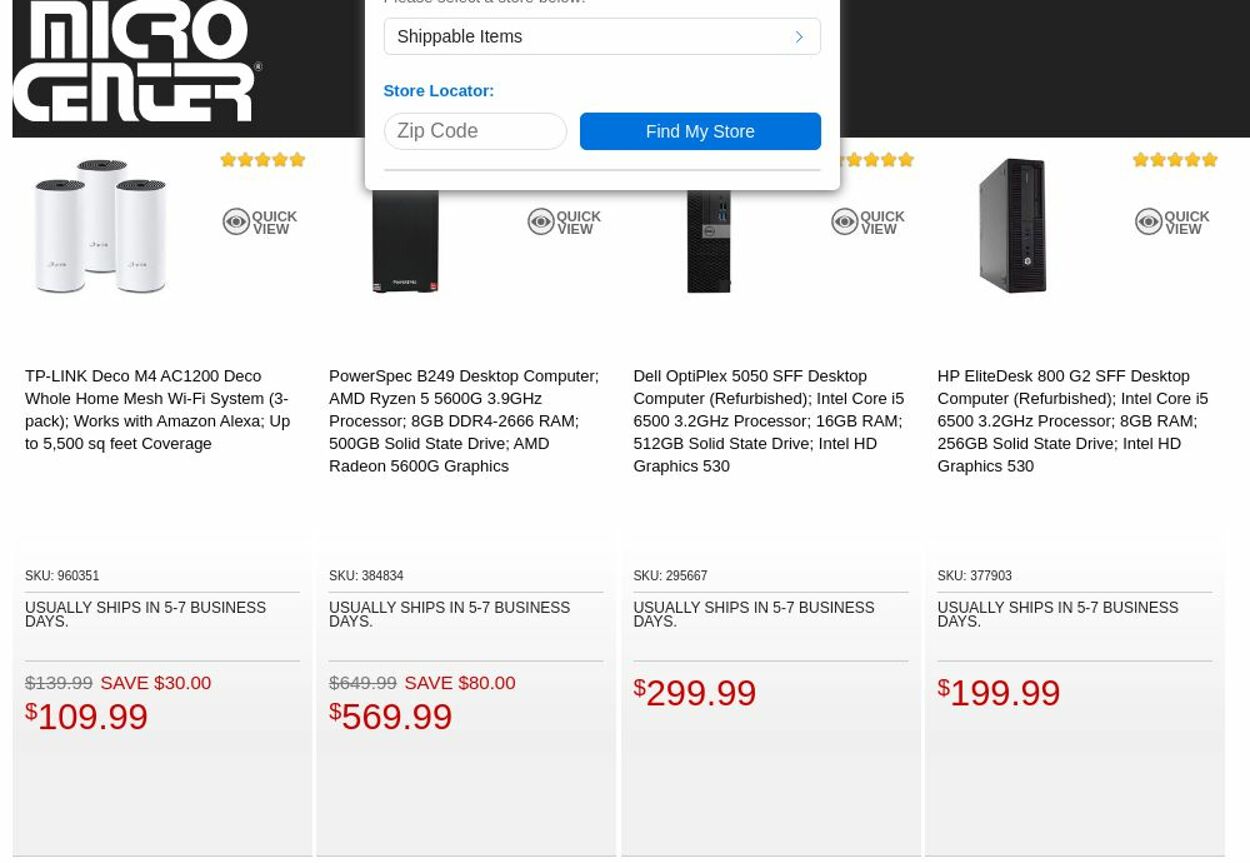The image depicts a section of the Micro Center website. 

**Top left:** The page header features a solid black background with the text "Micro Center" in white.

**Top center:** A pop-up notification displays various options, including "Shipping Item," "Store Locator," "Zip Code," and "Find My Store." The "Find My Store" button is prominently highlighted in blue.

**Main section:** The main page showcases four products each with a 5-star rating depicted in yellow at the top right corner. Directly below each rating, there is a "Quick View" button for a closer look at the product.

**Leftmost product:**
- **Title:** TP-Link Deco M4 AC1200 Whole Home Mesh Wi-Fi System 3-Pack
- **Compatibility:** Works with Amazon Alexa
- **Coverage:** Up to 5,000 square feet
- **Appearance:** Three white mesh units
- **Shipping:** Usually ships in 5-7 business days
- **Price:** Originally $119.99, now $109.99, saving $38

**Second product from the left:**
- **Title:** PowerSpec B249 Desktop Computer
- **Specifications:**
  - AMD Ryzen 5 5600G 3.9GHz Processor
  - 8GB DDR4-2666 RAM
  - 500GB SSD Drive
  - AMD Radeon 5600G Graphics
- **Appearance:** Black
- **Price:** Originally $649.99, now $569.99, saving $80

**Third product:**
- **Title:** Dell Optiplex 5050 SFF Desktop Computer (Refurbished)
- **Specifications:**
  - Intel Core i5 6500 3.2GHz Processor
  - 16GB RAM
  - 512GB SSD Drive
  - Intel HD Graphics 530
- **Price:** $299.99

**Rightmost product:**
- **Title:** HP EliteDesk 800 G2 SFF Desktop Computer (Refurbished)
- **Specifications:**
  - Intel Core i5 6500 3.2GHz Processor
  - 8GB RAM
  - 256GB SSD Drive
  - Intel HD Graphics 530
- **Price:** $199.99